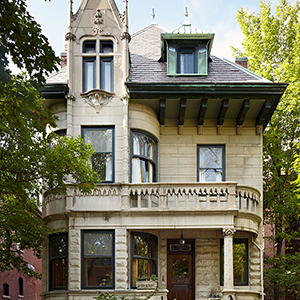This square photograph captures an old-style, two-story stone house made of beige-colored stone with a cream tint. The house features a hipped roof adorned with dark shingles, and there's a partly sunny sky with white clouds above. Surrounding the house are trees, with darker green leaves on the left and lighter ones on the right, giving it a quaint, natural frame. 

On the house's left side, there are three windows arranged vertically: one on the ground floor, one on the upper level, and a decorative window on the attic level. There is a prominent wooden door located in the middle lower section, flanked by a walkway with posts leading up to it. 

A notable feature is the upper level's walk-out area, enclosed by a railing. Behind this railing, on the right side, another glass window can be seen. The middle floor also has a mint-colored frame around one of the upper windows that slightly juts out, adding a touch of character to the structure. The house also hints at older architectural details with miniature statues perched on the pointed top of the left section, contributing to the building's distinct aged charm.